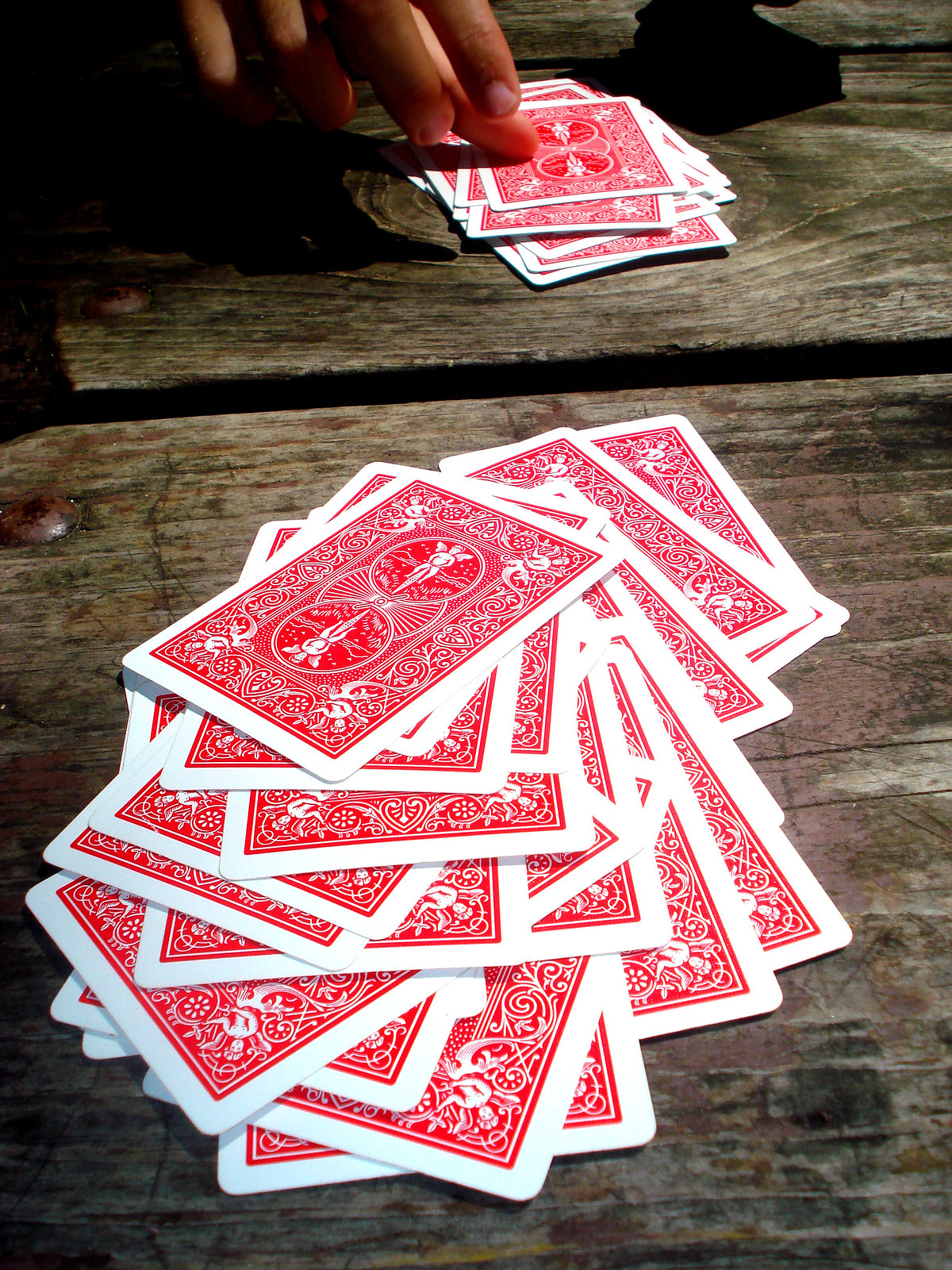In the photograph, a hand is seen resting atop a wooden table which is light brown in color. The table has a rustic appearance, featuring a notable detail in the form of a rusted nail or bolt embedded in it; this element is positioned slightly to the left of the center. The surface of the table is divided by a visible seam running between two wooden planks.

Scattered across the table are approximately 20 playing cards, all placed facedown. These cards have a distinctive red backing with a white border. Towards the top of the image, a white hand is seen gripping a smaller subset of the cards, holding them together in a stack of around 10.

In the top right corner of the frame, a black object is partially visible, while a hint of black appears in the top left corner as well. The rest of the image is devoid of other significant elements, with no additional people or text present, keeping the focus on the wooden table and the playing cards.